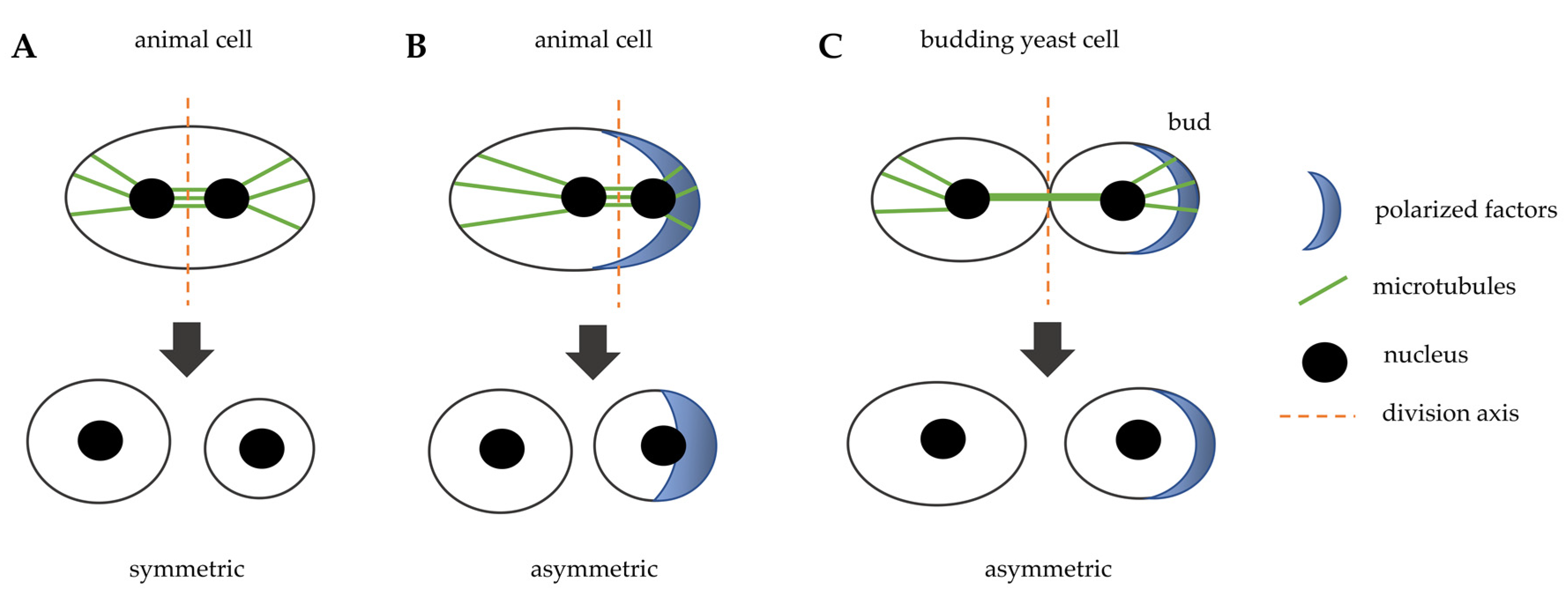The image is a scientific diagram with three sections labeled A, B, and C on a solid white background, illustrating different types of cell division. 

Section A, labeled "animal cell," depicts a single oval with colored and black dots and small green lines extending outward from the center. A thick black arrow points downward to two circles of different sizes with black centers, illustrating symmetric division. Below this, it is labeled "symmetric."

Section B, also labeled "animal cell," shows another oval where part of the edge is shaded in blue. A thick black arrow descends to two more circles with black centers, one of which is partially shaded blue, representing asymmetric division. This is labeled "asymmetric."

Section C, titled "budding yeast cell," consists of an oval shape and a circle, with one side shaded blue and labeled "bud." A dotted dashed line separates the two shapes. A thick black arrow points downward to another oval and circle, indicating asymmetrical division. This section also includes a crescent-shaped area shaded in blue labeled "polarized factors." Adjacent text indicates that the green lines represent microtubules, the colored and black circle is the nucleus, and the dashed line marks the division axis.

Overall, the diagram provides a detailed comparison of symmetric and asymmetric division in animal cells and demonstrates the budding process in yeast cells.